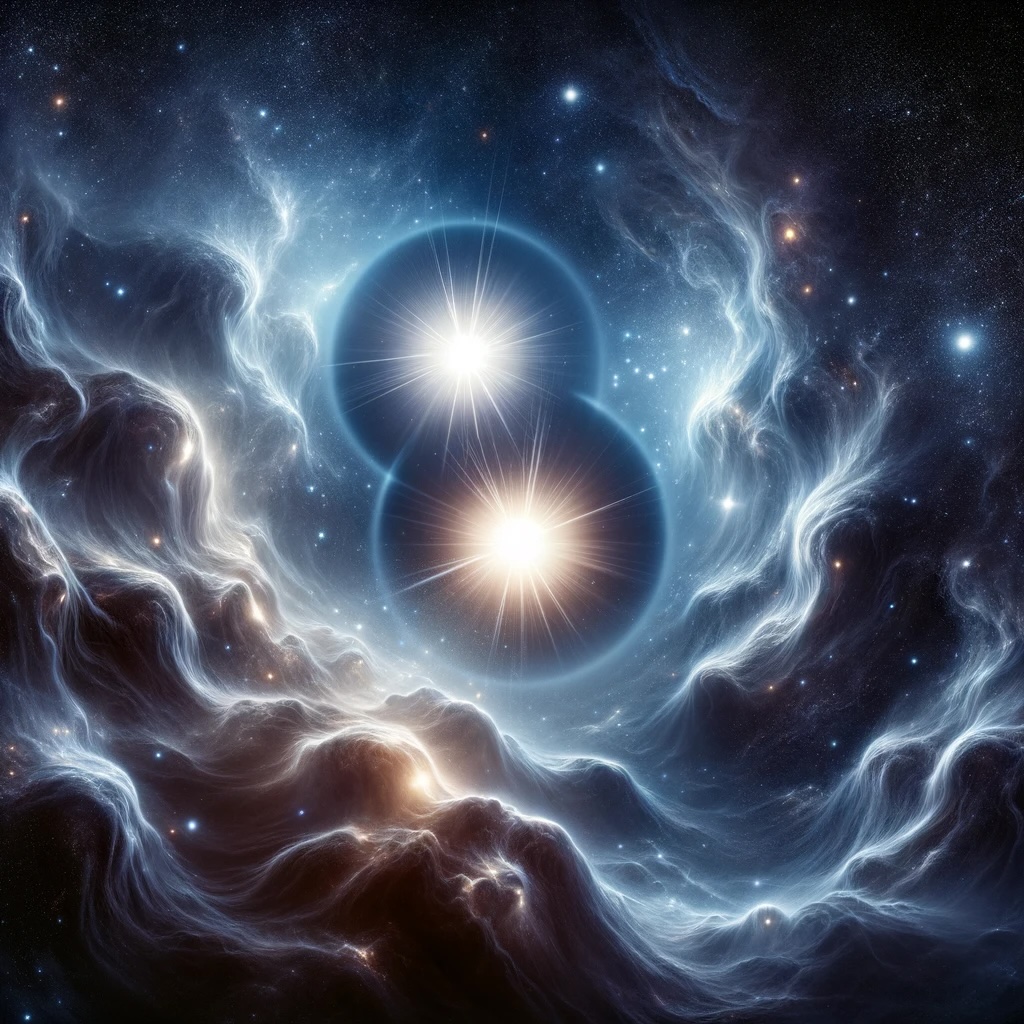This image appears to be an AI-generated artistic representation of a captivating space scene. Dominating the center, two luminous stars, aligned vertically, each surrounded by a distinct halo, together appear reminiscent of the number eight. These halos create an impression of overlapping orbs or spheres, one star glowing bright silver and the other with an auburn hue. Encasing these celestial bodies is a swirling, cloud-like nebula, forming an oval shape that envelopes the stars. The nebula's texture resembles smoke or water, filled with various smaller stars and space objects, showcasing a palette of blue and soft yellow tones. The overall effect is an ethereal depiction of an intergalactic phenomenon, possibly hinting at a solar eclipse or a unique astronomical event within a galaxy.